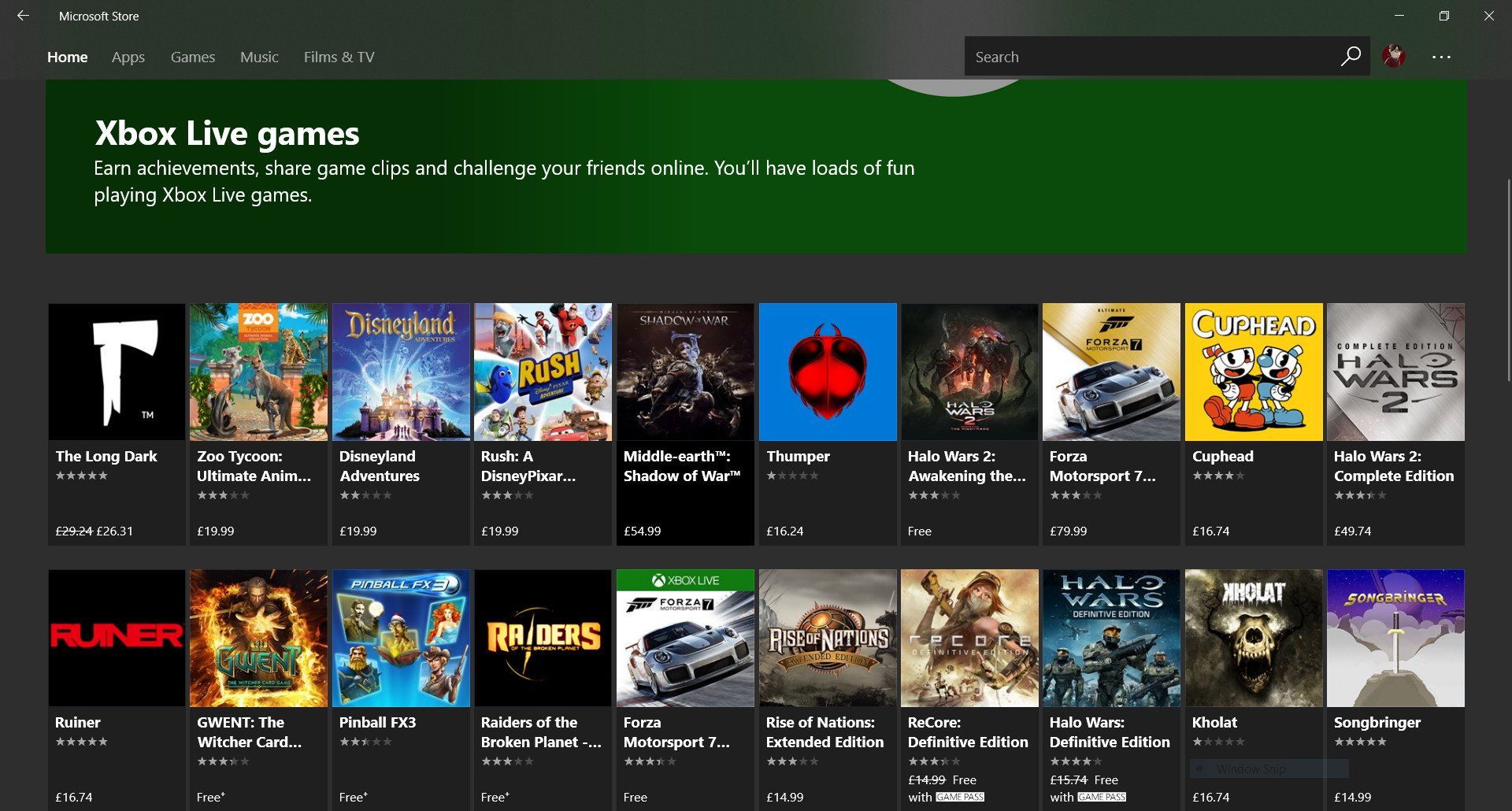The image appears to be a screenshot of the Microsoft Store interface. The window has a distinct gray-green background that's slightly blurry. At the very top, the title bar reads "Microsoft Store" and includes the standard window control buttons—minimize, maximize, and close—on the right-hand side. On the left side of the title bar, there's a navigation arrow pointing left.

Below the title bar, there's a menu bar featuring navigation options: Home, Apps, Games, Music, Film, and TV. A search bar, identifiable by a magnifying glass icon, is positioned towards the center of the interface. To the far right, there's a user avatar indicating the currently signed-in user, along with a three-dot (ellipses) icon for accessing more options and settings.

A prominent banner below the menu highlights Xbox Live Games, encouraging users to earn achievements, share clips, and challenge friends online, promising loads of fun. Underneath this banner, there are two rows displaying a total of ten game titles. The games include "The Long Dark," "Zoo Tycoon," "Disneyland Adventures," "Rush: A Disney Pixar Adventure," "Middle-earth: Shadow of War," "Thumper," and "Halo Wars 2," among others. This selection showcases a variety of genres and popular titles available in the store.